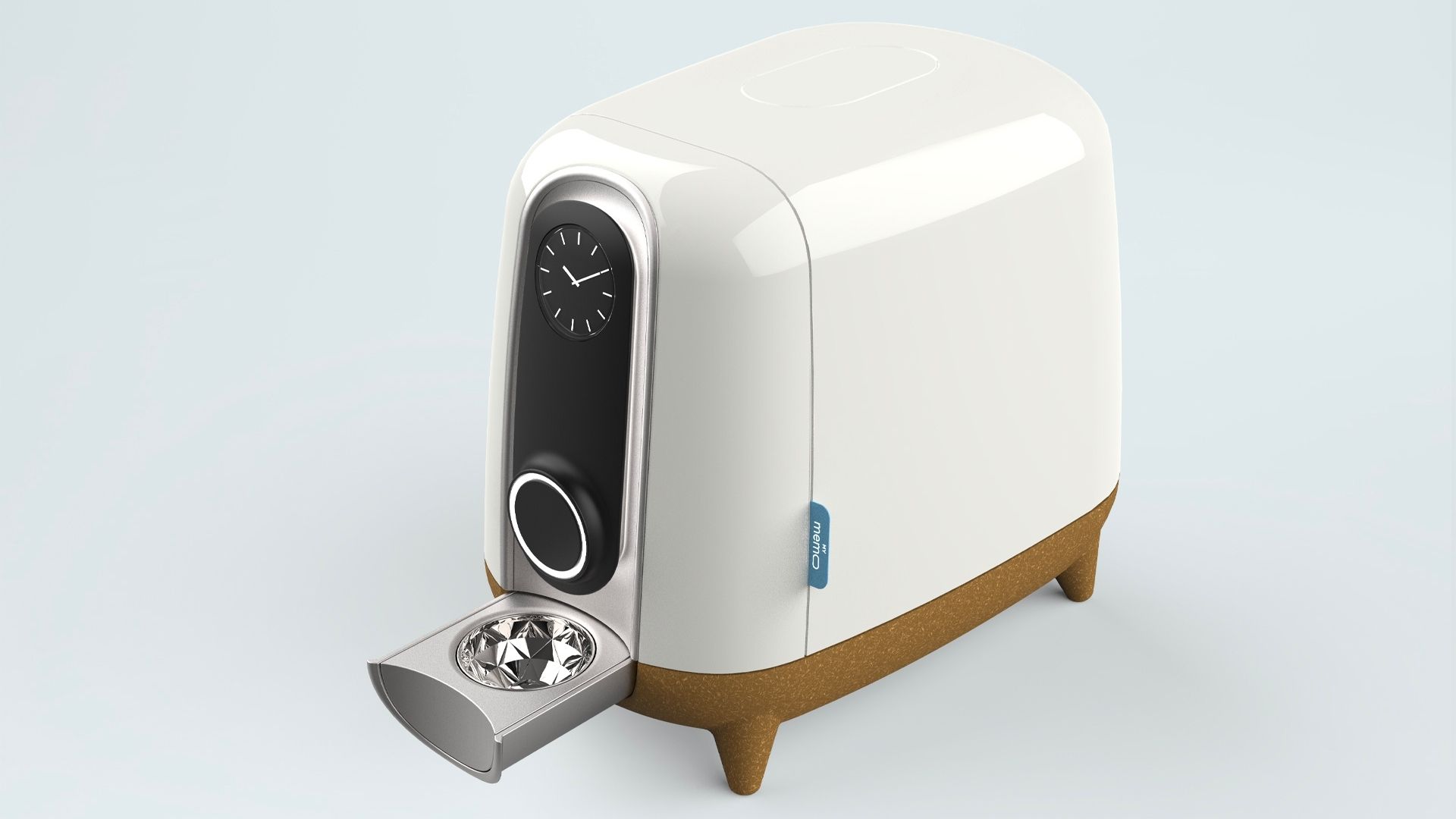The image depicts a high-tech, white, rectangular device that superficially resembles a toaster but lacks the traditional bread slots. The sophisticated device features a black oval-shaped panel on the top, which houses a clock with lines instead of numbers. Below the clock is a raised button encircled by a white ring. There's also a small tray or dispenser at the bottom, distinguished by a shiny, diamond-like glass hole. The device stands on a brown base with four rounded legs, giving it an elevated appearance. The background of the image is a minimalist gray field, highlighting the advanced and elegant design of the mysterious appliance.